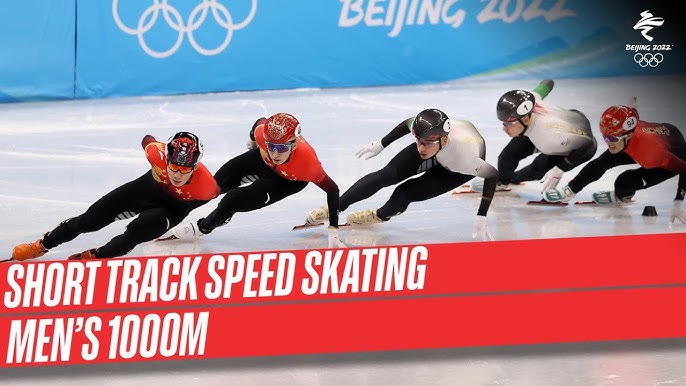The image depicts a high-action moment from an Olympic short track speed skating event featuring five male skaters navigating a sharp turn in unison, almost parallel to the ice. Leading the pack is a skater in a red jacket, black pants, and red speed skates, distinguished by his black helmet adorned with red markings. Close behind is another skater in a similar red jacket, but with a predominantly red helmet with yellow decorations. The third and fourth skaters sport black pants and white jackets, their black helmets marked with white ovals on the sides. The fifth skater mirrors the second in his red jacket and black pants. Their helmets vary in color and design, featuring numbers and multicolored patterns including black, red, white, and gold. All five skaters, dressed in white gloves, are so close to the ice that their hands touch it for balance. The rink's blue walls prominently display the Beijing 2022 logo with the five Olympic rings. This logo also appears in the upper right corner of the image. Overlaying the bottom of the image are two red bars, the top bar labeled "SHORT TRACK SPEED SKATING," and the bottom bar noting, "Men's 1,000 meters."